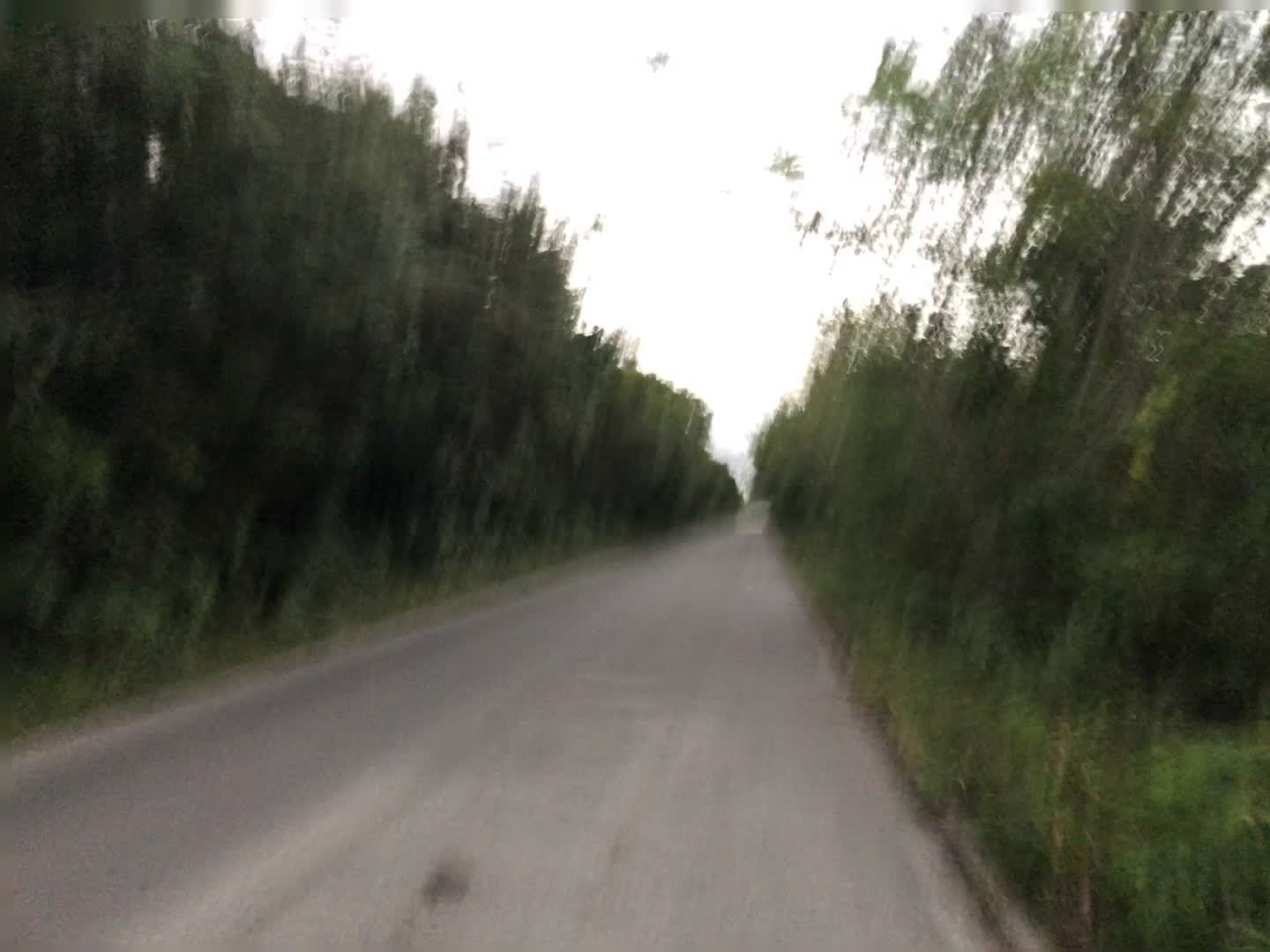This image depicts a blurry photograph of a narrow two-lane highway, possibly a wide path. The road, constructed of gray concrete, features a faintly visible center line and distinct white lines marking the edges. Lush wild grass lines both sides of the pavement, leading up to a dense array of wild trees. The sky above is exceedingly bright, almost bleached out, making it difficult to discern specific details. The overall blurriness suggests the camera might have been in motion when the shot was taken. In the middle of the road, there is some darker texture, though it remains unclear whether it represents an object in motion or a characteristic of the road itself. Additionally, a few birds can be seen flying out of the trees, their shadowy forms barely distinguishable against the bright backdrop.